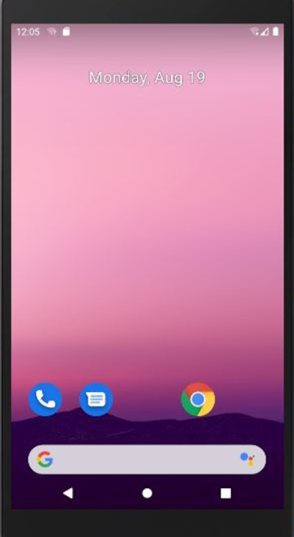The image depicts a cell phone screen with various visual elements and icons. 

At the top left corner, the time "12:05" is displayed in white text. On the top right, icons for Wi-Fi or data, signal bars, and a full battery are visible. The date "Monday, August 19th" is centered at the top of the screen, also in white text.

The screen's wallpaper features a gradient of colors, starting with dark purple at the bottom resembling hills, transitioning to lighter shades of purple, and then to various shades of pink as it moves upward, mimicking a pink-purple sunrise or sunset. The colors blend from light purple to dark pink, becoming progressively lighter until the top of the screen, which is the lightest shade of pink.

At the bottom of the screen, there are app icons for Phone, Messages, and Google, situated above a Google search bar. Below this bar are navigation icons for the phone, including a back button, a home button represented by a circle, and a square for recent apps.

All the text and icons are white, contrasting against the colorful background. Notably, the image appears to have a thick black border around it, suggesting it may have been superimposed onto a black background. Additionally, the resolution of the image is quite low, impacting the overall clarity and sharpness of the visual elements.